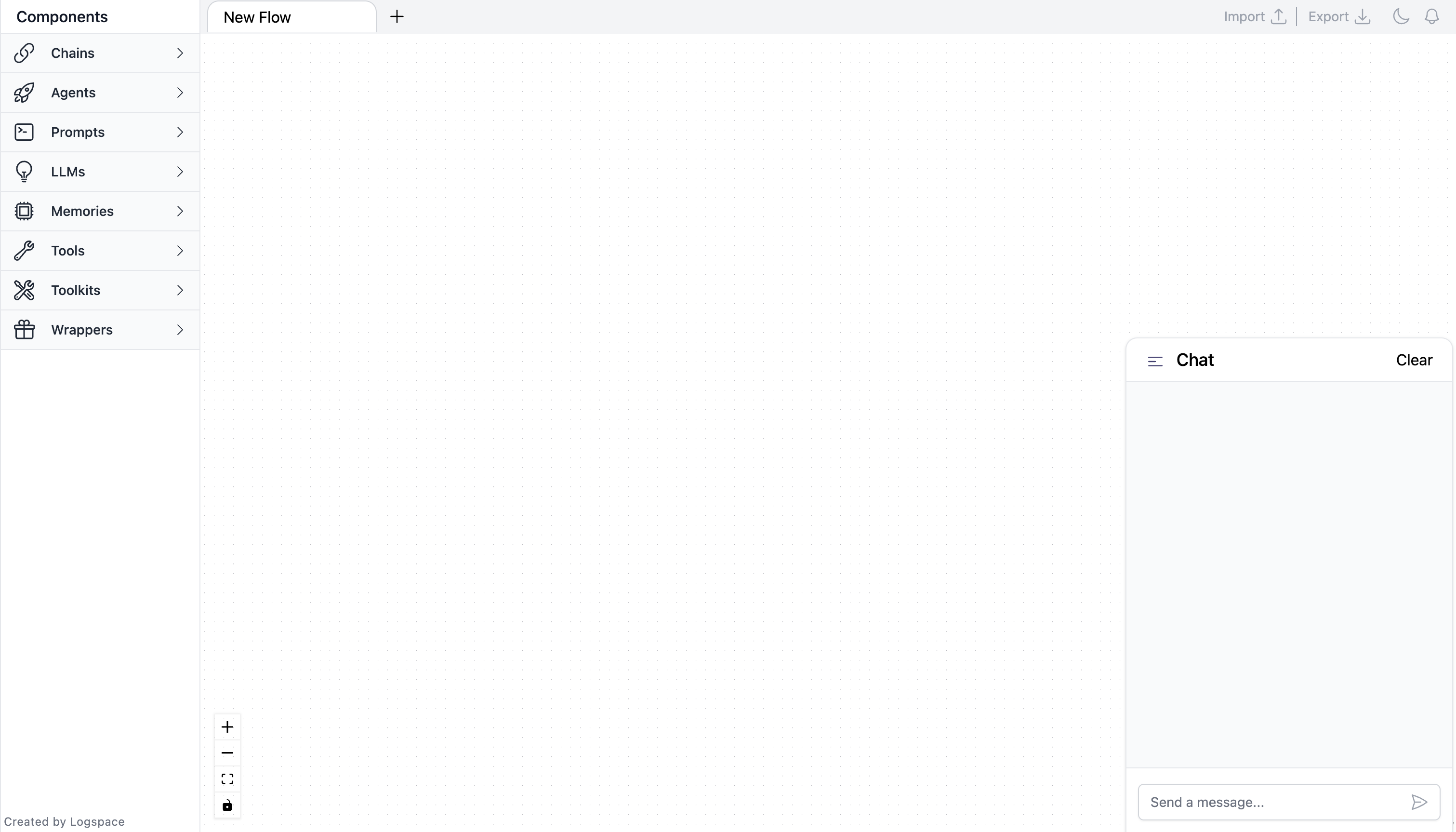**Detailed Caption:**

The image depicts a computer interface window with a predominantly white background. At the top left corner, the word "Components" is prominently displayed. Adjacent to this, extending horizontally to the right edge of the image, is a gray rectangular bar. This bar contains various interactive elements. On the left side of the bar, there is a tab labeled "New Flow" with a white background and black text. Next to this tab is a black plus icon. Moving further to the right, on the far end of the gray bar, there are several icons and options: an "Import" option with an upward arrow, an "Export" option with a downward arrow, a moon icon outlined in gray, and a bell icon also outlined in gray.

Beneath the "Components" text, there is a vertical list of options: "Chains," "Agent," "Prompts," "LLMs," "Memories," "Tools," "Toolkits," and "Wrappers," all written in black text. Each option is accompanied by a corresponding icon and a gray right arrow. Below this list, there is a substantial amount of white space. At the bottom of this section, there is a small text that reads "Created by Log Space" in gray.

The lower portion of the window features a large white space with a pattern of gray dots scattered across it. In the bottom left corner of this area, there is a vertical stack of icons enclosed in white squares with gray outlines. These icons include a plus icon, a minus icon, a full-screen icon, and a lock icon. On the bottom right side of the window, there is a chat box labeled "Chat" in the top left corner. The top right corner of the chat box has a "Clear" option. Directly beneath this, a gray rectangle is visible. Below it, there is a white horizontally-oriented rectangle with rounded corners, displaying the placeholder text "Send a message..." in gray, accompanied by a right-pointing arrow.